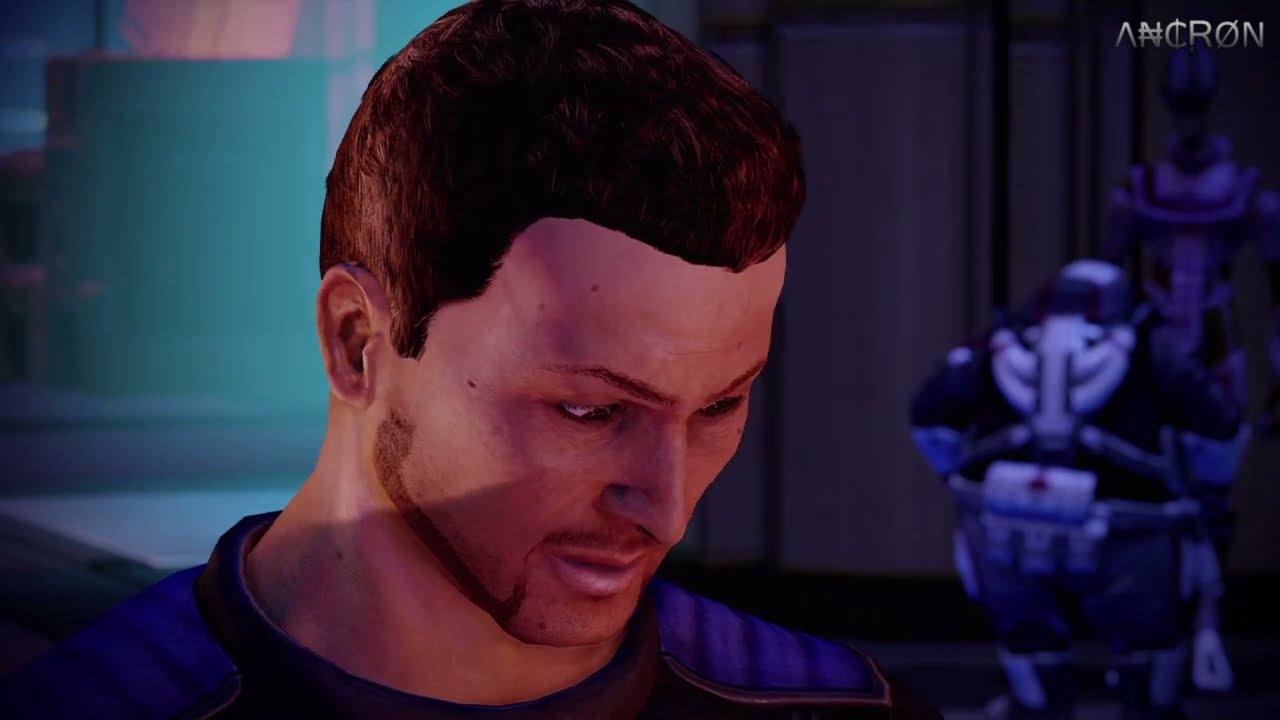The image appears to be a still from a video game, featuring a relatively lifelike depiction of a man with short, reddish-brown hair and a sharp, pointy nose. He has a small mustache and a wiry beard that lines his jaw, forming a short, shaved goatee at the lower part of his chin. His eyebrows, matching his hair color, are slightly tilted inward, suggesting he is looking at something on the ground. The man, shown from his shoulders up, is wearing a black top accented with bright blue and dark blue stripes on the shoulders, which end in a square shape indicative of shoulder pads. His head is slightly turned towards his right, providing a nearly side profile view, and he seems to be looking downward towards the center lower part of the frame. 

Behind him, the background is a gradient, shifting from green on the left to purple with some black lines on the right. In front of the purple background stands a blurry, black robot with a white face. The robot appears somewhat fat and is equipped with a belt-like accessory that has a white pouch positioned in front of its belly. In the top right corner of the image, the letters "A-N-C-R-O-N" are visible, adding a possible context or brand element to the scene.